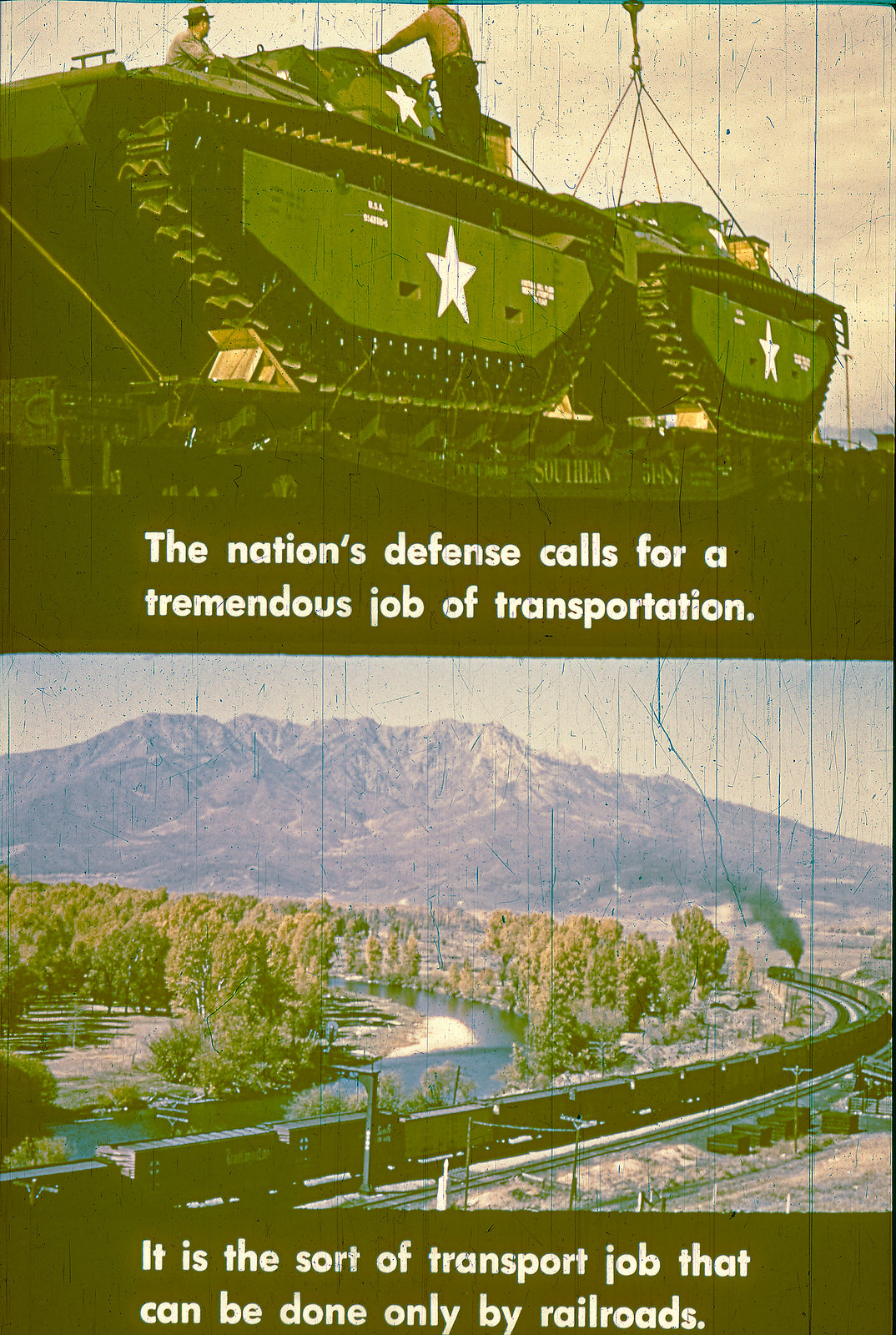The image is divided into two sections, each featuring a photograph. The top half displays two military tanks on a flat train car, with two engineers working on them. The tanks are predominantly green with a white star on their armor, positioned between the tracks and beside a hatch area. The rear tank is anchored with construction wires. Below this, a dark-colored banner with white letters reads, "The nation's defense calls for a tremendous job of transportation." The bottom half of the image depicts a snowy forest landscape with a river running through it. A train, laden with numerous cars, navigates the scene from the bottom left, curving to the right, and then back to the left towards a mountainous background. Below this photo, another banner states, "It is the sort of transport job that can be done only by railroads."